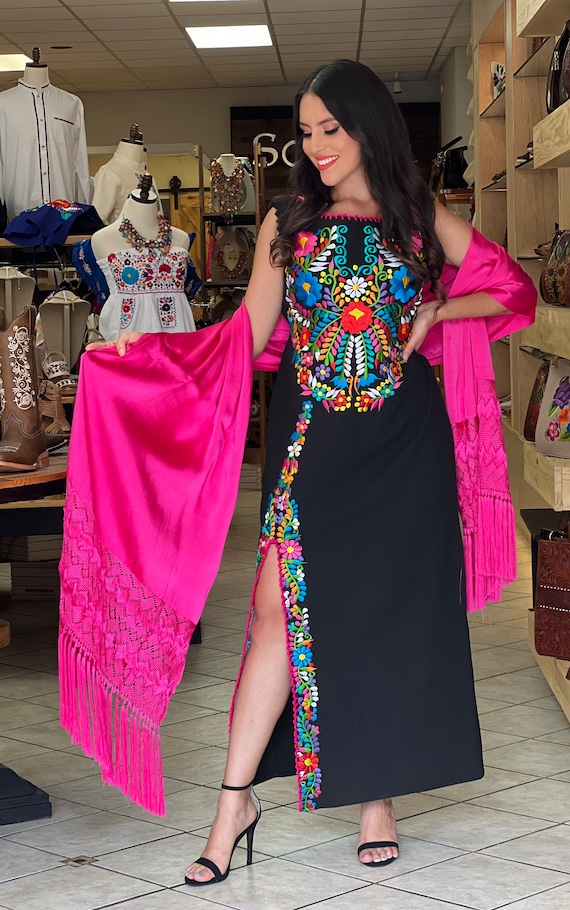This image captures a lovely, young woman in a store, elegantly modeling an outfit. She is dressed in a long, black dress embellished with elaborate, multicolored embroidery, including blue, yellow, green, and purple floral designs. The dress features a split up to the knee, revealing her black high-heeled pumps. Draped around her shoulders is a bright pink satin shawl adorned with embroidery and tassels, which she holds delicately in her right hand. The woman has long, dark hair with wavy tips, dark eyes, and she is smiling while looking down, revealing her bright, white teeth and red lipstick. Behind her, the store displays a variety of items including mannequins dressed in tops, cowboy boots, and racks with purses and various shoes. The floor is a white tile, and the ceiling consists of drop panels with fluorescent lighting, all contributing to the shop's busy atmosphere.